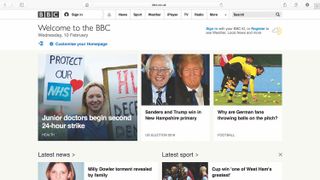The homepage of the BBC website prominently features a welcoming heading that reads "Welcome to the BBC." The layout is visually engaging, with a total of five photos, albeit two are partially visible. The top section showcases three distinct images: 

1. On the left, there is a photo of a woman holding a sign that reads "Protect our NHS," accompanied by a headline stating, "Junior Doctors Begin Second 24-Hour Strike."
2. The center of the page displays a juxtaposition of Bernie Sanders on the left and former President Trump on the right.
3. To the right, there is an image of German soccer players donning yellow and black uniforms.

At the bottom of the page, there are two additional images that are partially cut off and therefore not fully discernible. The fourth picture, located at the bottom left of the screen, and the fifth picture, situated at the bottom right, both remain unidentified due to their obscured nature.